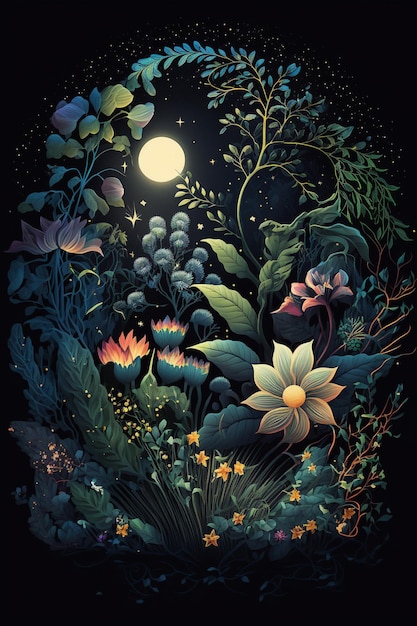This is a contemporary, digitally drawn image of a nighttime forest scene. The backdrop is black, highlighting the moon nestled in the top left corner, casting a delicate yellow glow. Stars are scattered across the upper portion of the image, enhancing the nocturnal atmosphere. The foreground is a vibrant collection of natural elements arranged in an oval shape. This includes a multitude of flowers in various colors—yellow daffodils, orange blossoms, touches of pink, and blue tones—densely packed together. Greenery in diverse shades, from vivid greens to greenish-blues and purples, surrounds the floral arrangement. The plants vary in size and type, with some large, draping leaves and others resembling sprouts or vines. The perspective of the artwork appears to ground the viewer, looking up at the moon through this dense, colorful array of flora. The detailed and carefully composed scene evokes a sense of tranquil beauty, suggesting it could be a striking piece in a graphic designer's portfolio or a poster suitable for a teenager’s room.